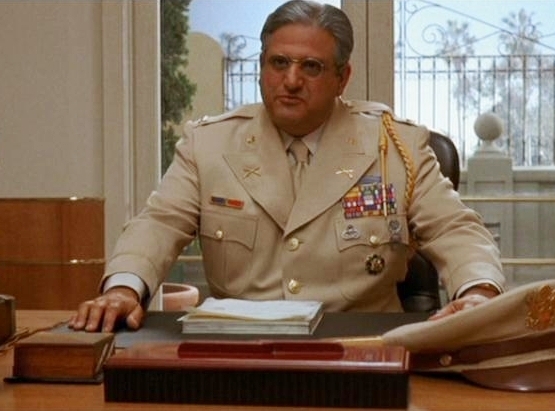This is a horizontal rectangular photograph featuring a stern-looking military officer of an unspecified branch of service, seated at a desk. The officer is adorned in a khaki colored uniform, comprising a jacket, shirt, and tie, complemented by a white shirt beneath. His uniform is heavily decorated with numerous medals, pins, stars, and a distinctive braided gold cord draped over his left shoulder, signifying a high rank and commendations. The officer, who has short, dark brown hair, is captured in a somber, serious pose, not smiling, and wearing glasses. 

On the desk, there is a collection of items, including storage boxes, a stack of papers, a desk blotter, and the officer’s matching hat, which is beige with a brown strap. The desk is positioned in front of a window, through which a couple of trees and a clear sky can be seen. Additionally, there is a view of two doors leading to a small balcony adorned with a decorative wrought iron gate. The officer is seated in a brown chair, adding to the formal and disciplined atmosphere conveyed in the image.